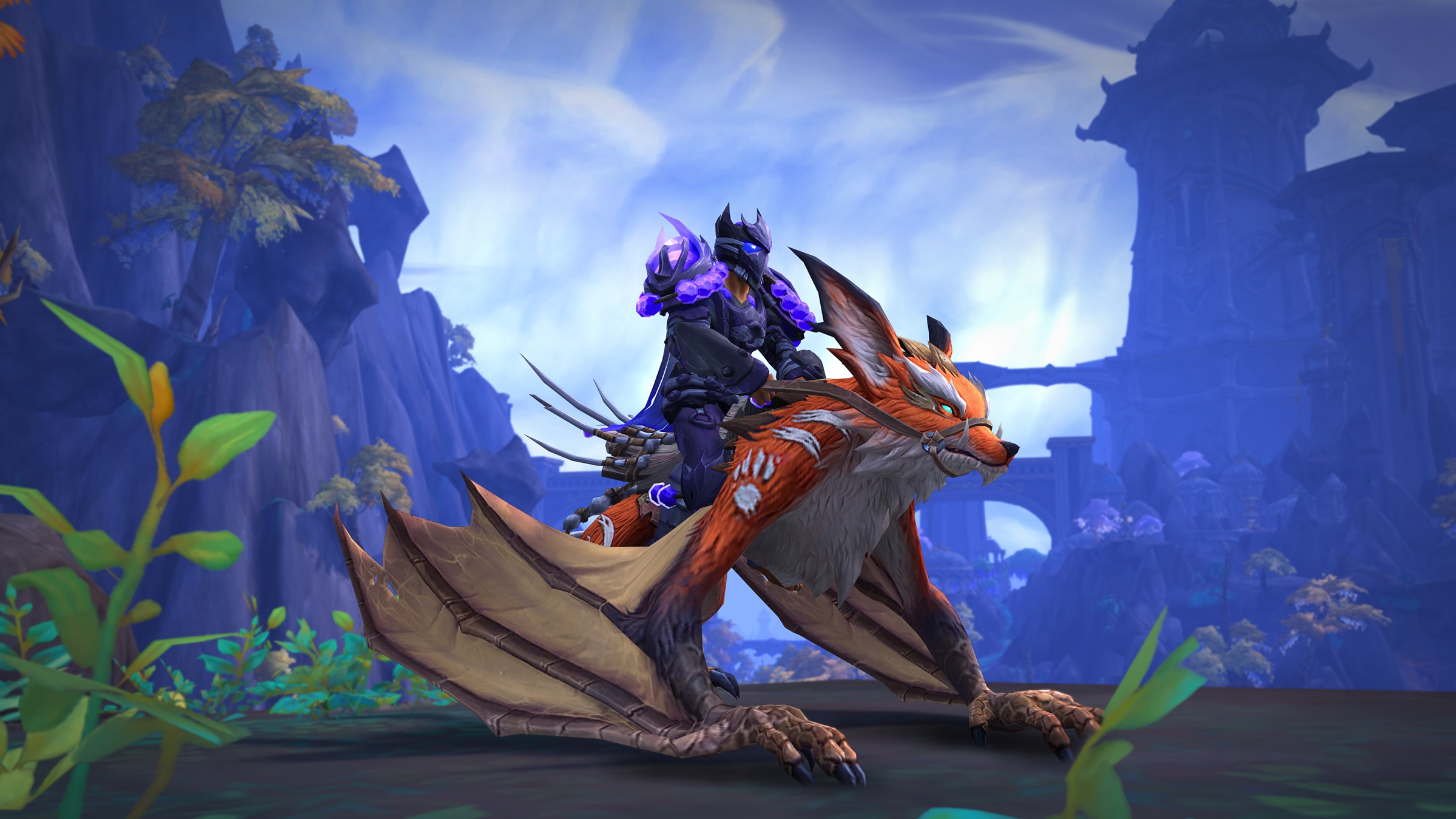The image is a highly detailed screenshot from a computer game, potentially reminiscent of the styles seen in games like Transformers or World of Warcraft. It features a hybrid creature with the body and face resembling a fox but combined with bat-like features. The creature is predominantly orange with large, foxy ears and white fur, but its limbs end in brown claws, and it has expansive bat wings attached to its paws.

Mounted on this fantastical creature is a character clad in intricate, dark armor with purple accents. The armor appears almost metallic, covering the whole body, including a mask and helmet that obscure the rider's face. The knightly figure is seated on a saddle on the creature's back, giving the impression of a ready-for-battle stance.

The background is enveloped in a purplish hue and includes various environmental details such as palm trees, cliffs, grassy areas, and towering buildings that could be castle-like structures. The ground is rocky, adding to the fantastical and adventurous atmosphere of the scene. The image is rectangular, with the width being twice the height, capturing an immersive and detailed fantasy setting.